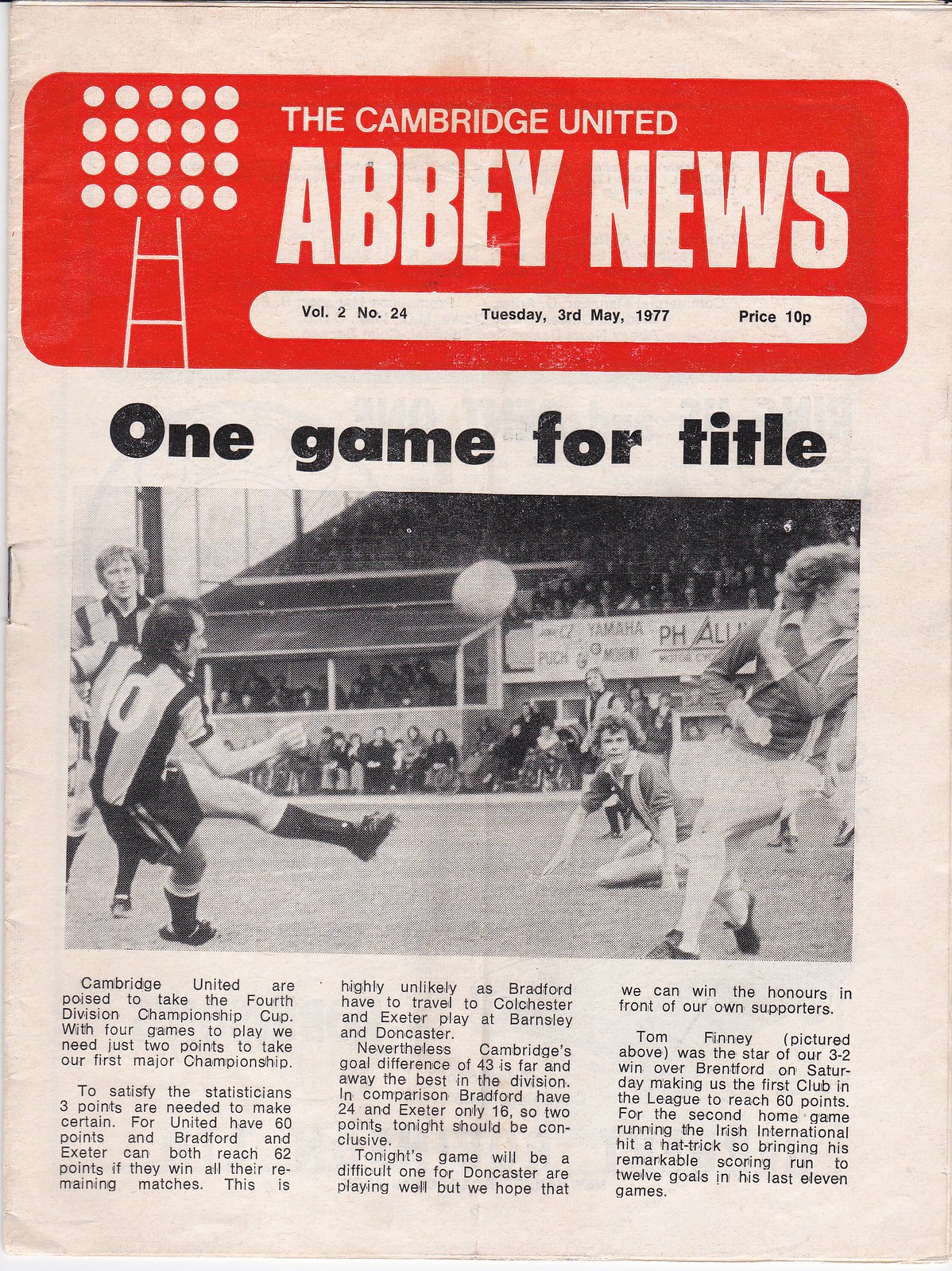The image is a vertical rectangular front cover of a publication, likely a magazine or newspaper, that provides information about a soccer team. At the top, a large red banner reads "The Cambridge United Abbey News" with "the Cambridge United" in small letters and "Abbey News" in larger letters. To the left of this banner, white lights, similar to those illuminating a playing field, are depicted. Underneath "Abbey News," a white oval displays the date and publication details: "volume 2, number 24, Tuesday, 3rd May, 1977, price, 10p." 

Dominating the front page, a headline in bold black letters reads "One Game for Title." Below the headline is a black and white photograph capturing two soccer teams in action, with the ball suspended in mid-air. One player, wearing dark shorts, has their left leg kicked up, implying they have just kicked the ball. The scene is set against a backdrop of spectator stands. Additionally, text within the cover mentions that Cambridge United is on the brink of winning the Fourth Division Championship Cup with just two points needed from four remaining games to secure their first major title. The cover emits a sense of anticipation and excitement, typical of a program handed out at soccer games.